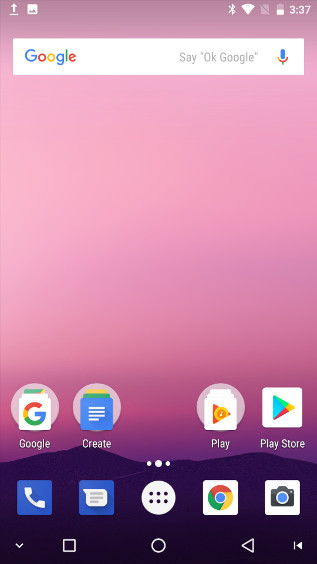A vivid display of an Android device's home screen is captured in a photo that appears to be of an older version of Android, though the exact iteration is uncertain. On the upper right-hand corner, the time is displayed, accompanied by battery, Bluetooth, and Wi-Fi indicators, among other status icons. The upper left hosts additional, less familiar UI elements. The background boasts a striking gradient, transitioning from pink to purple.

Dominating the top center of the screen is the ubiquitous Google search bar, which offers the functionality to either type a query or use the small blue microphone icon to activate voice search with "OK Google." 

The bottom section of the screen is a hub of activity, populated with a variety of app icons including Google Chrome, Camera, Play Store, and Google Play. There are also icons for essential functions such as the Phone and Messages apps. Situated at the very bottom of the interface are the navigation controls, featuring buttons to return to the home screen, close apps, and access additional controls.